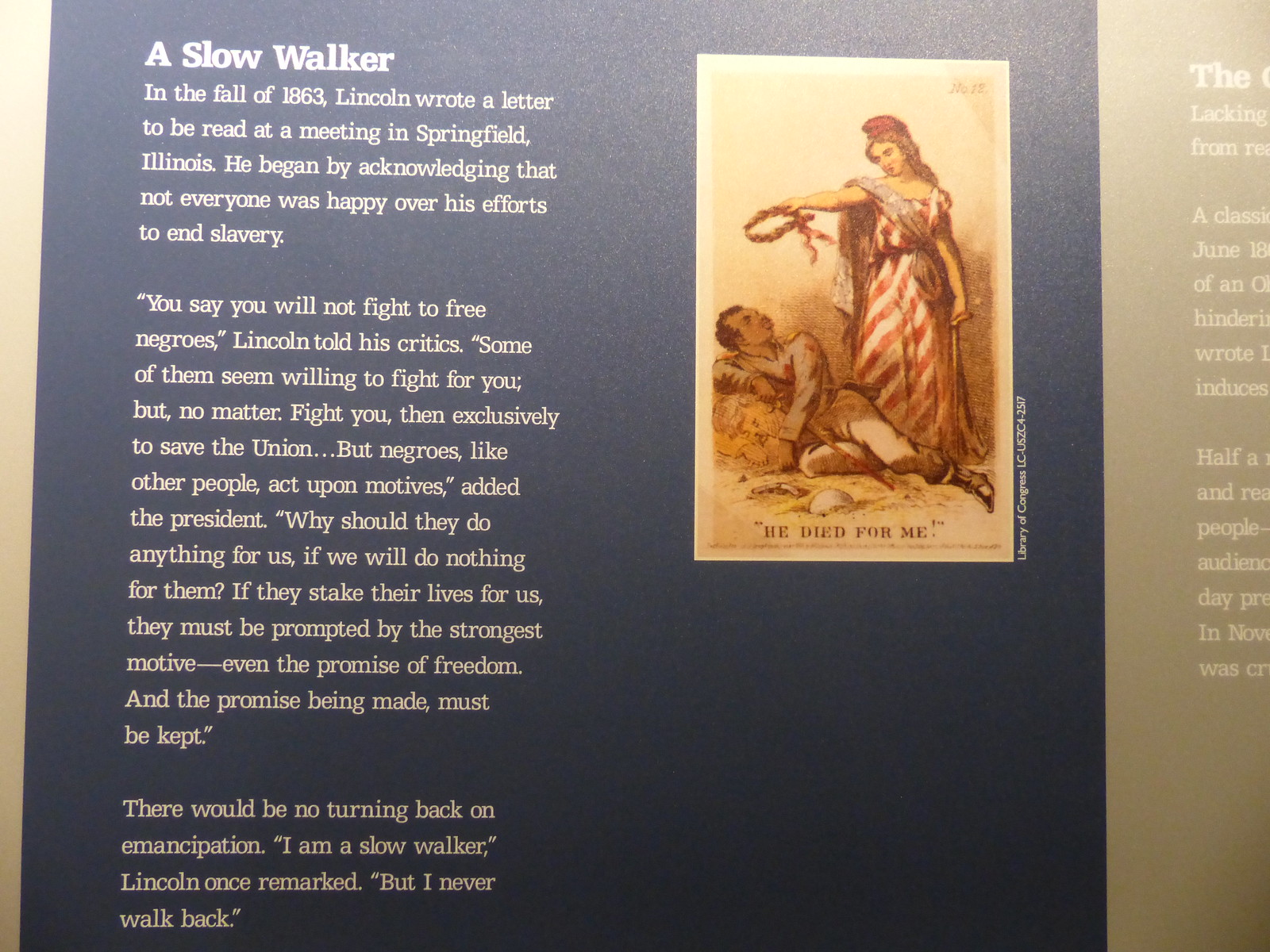The image depicts what appears to be a page from a book or an educational poster featuring detailed historical text and an accompanying illustration. The central focus is on a blue-columned section with white text that reads "A slow walker." This section quotes an 1863 letter by Abraham Lincoln addressing critics of his anti-slavery efforts, where Lincoln acknowledges the motive behind freeing the Negroes and emphasizes the irrevocability of emancipation with the words, "If they stake their lives for us, they must be prompted by the strongest motive, even the promise of freedom." An illustration to the right of this text shows a white woman standing over a seated, possibly collapsing, black man. The woman appears to be holding an indistinct object, resembling a rounded wreath or possibly a hunter. The illustration is captioned with, "He died for me." This image is mostly centered, suggesting a formal, educational presentation, possibly as part of a book or a poster. The scene is sharply divided by a vertical crease, and there is an adjacent column with cut-off text on a brown background visible on the far right.